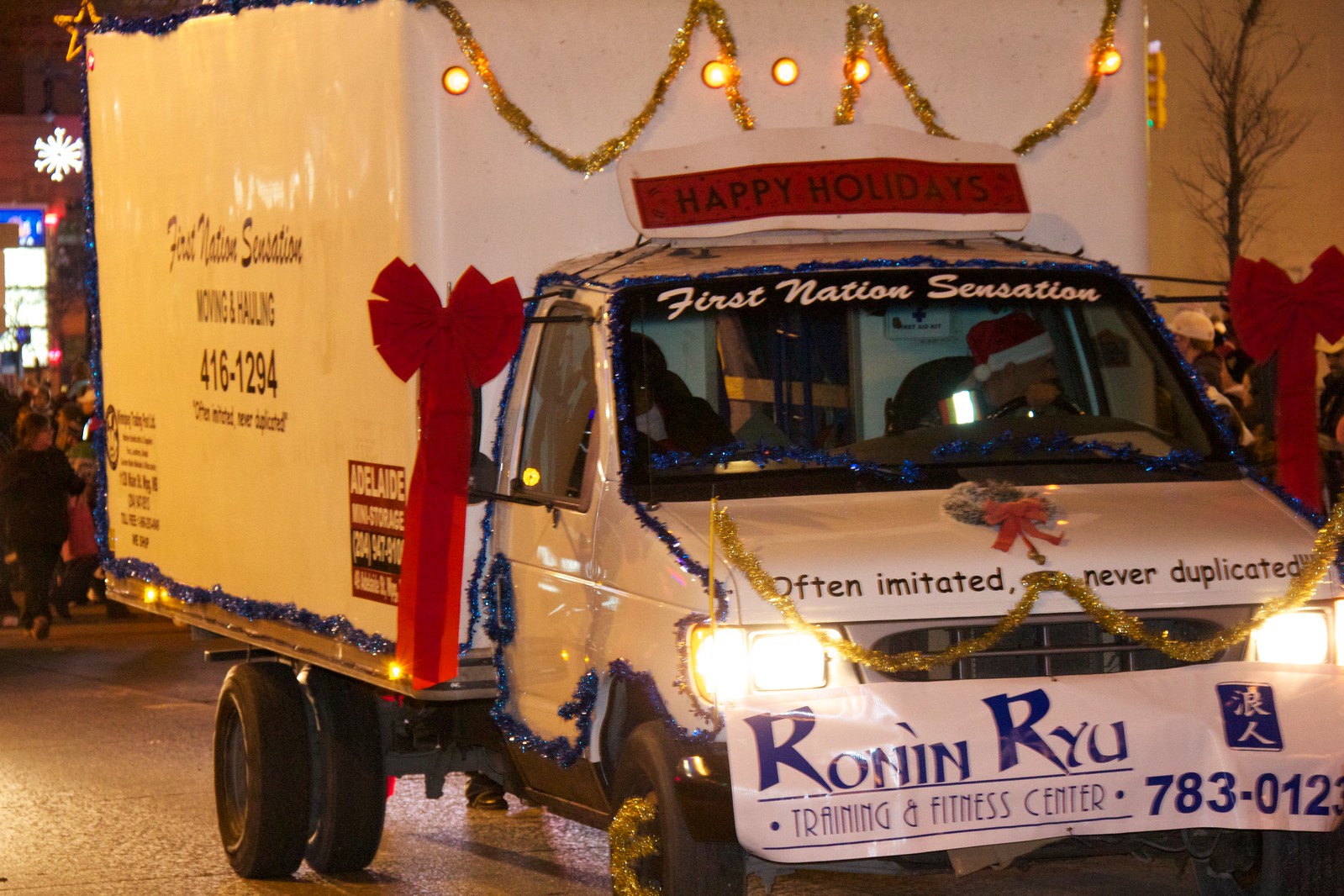The image features a semi-diagonal front view of a white box truck decorated in festive winter holiday decorations, prominently set against a nighttime outdoor backdrop. The truck is centrally positioned on an asphalt road typically used by cars. Elaborate holiday decor adorns the vehicle, including twinkling lights, tinsel, ribbons, garlands, and a large red bow. A banner reading "Happy Holidays" sits atop the truck bed roof, and another sign on the windshield reads "First Nation Sensation." The front bumper displays a wreath and bears the slogan "Often Imitated, Never Duplicated." The truck advertises Ronin Ryu Training and Fitness Center, with a phone number provided. The truck's hubcaps are wrapped in gold garland, contributing to the festive appearance. Inside the cab, two people can be seen, one wearing a Santa hat. In the background, a crowd of people is visible, adding to the holiday atmosphere. The truck itself features various colors, including gray, black, blue, red, gold, yellow, tan, and white.